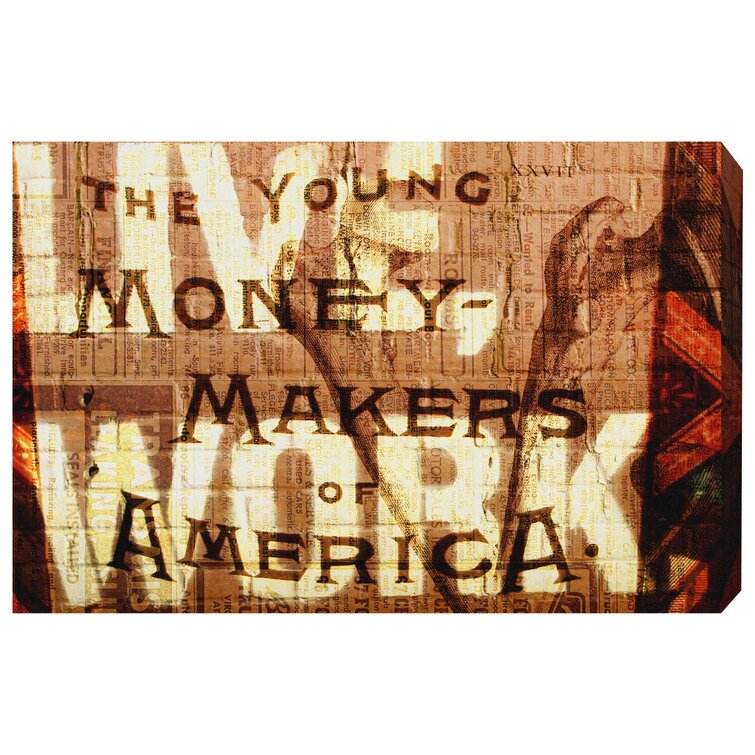The image is a photograph of an eye-catching mural painted on a brownish brick wall, possibly located inside or outside an office building. The mural prominently features the words "Live Work" in large, blocky, off-white letters. Overlaid in a smaller, dark brown, old-fashioned font is the phrase "The Young Moneymakers of America." The background bricks are light brown with various shades creating a sense of depth and shadow. Additionally, there is an artistic red V-shaped element in the middle of the mural, on the right-hand side of the image, contributing to its striking visual composition. The mural also includes vertical text and images that resemble painted fabric, adding to the overall complexity and appeal of the artwork.